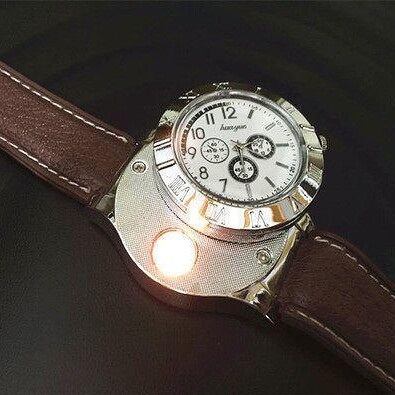This photograph captures an intricately detailed, exploded view of a wristwatch laid diagonally on a dark, natural background. The watch features a brown leather strap accentuated by light-colored stitching running along both edges. The metal face of the watch has been removed and is slightly off-center but still rests on top of its intended position, revealing the screws and interior components beneath.

The watch face is predominantly white and includes a unique numeral configuration; numbers from 7 to 12 are displayed, while the positions of the remaining hours are marked by simple metal rectangles. Additionally, three smaller dials are embedded within the face, likely indicating date, water-resistance, and perhaps other functionalities. The exterior bezel of the watch is adorned with Roman numerals, specifically highlighting the numbers 5, 6, 7, and 8 at the bottom, and 11 and 12 at the top, in alignment with the larger face numerals.

A knurled edge winder is visible on the watch's side, used to manually wind the mechanical components. Every element, from the detailed strap to the removed, slightly repositioned face, contributes to the photograph’s intricate and meticulous presentation.